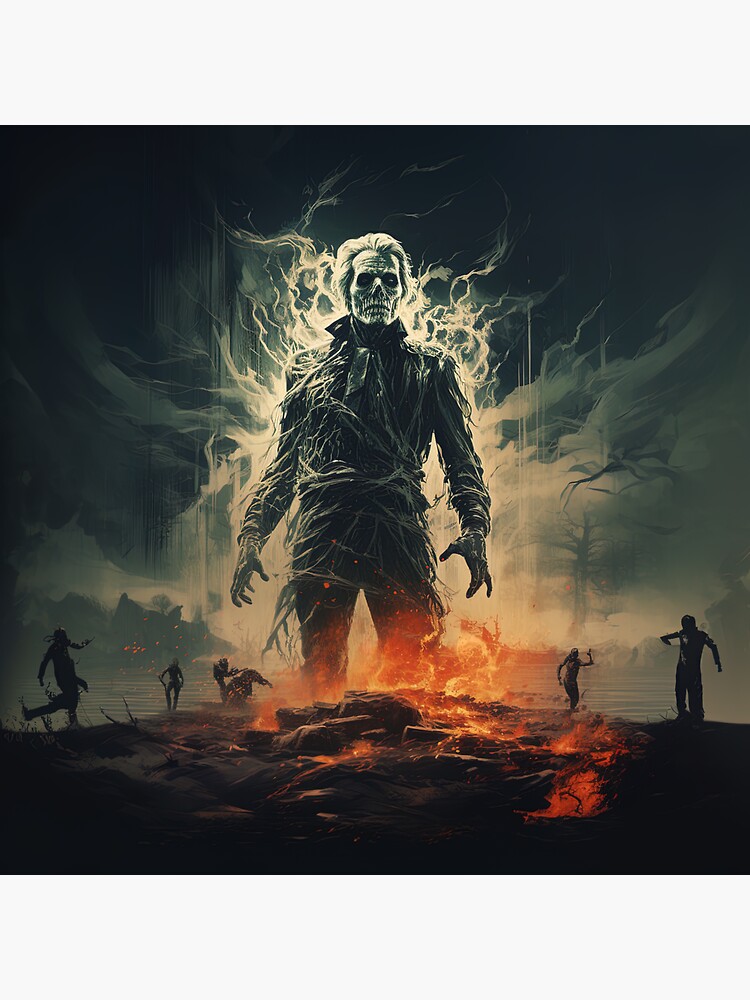In a dark, eerie scene reminiscent of a graphic novel, the image portrays a colossal zombie towering amidst a hellish landscape engulfed in flames and lava. The sky above is a mix of dark blue and black, adding to the overall spooky atmosphere. The giant zombie, about 60 feet tall, has a skeletal face with hair, strikingly similar to the Marvel character Ghost Rider, and is covered in twisted vines as if emerging from the earth. Orange flames and white steam or electrical arcs emanate menacingly from its body. Surrounding the central figure, several smaller zombies, some in the foreground and others in the background, stagger aimlessly towards the fire. The terrain is jagged and treacherous, with molten lava spilling forth where the giant zombie stands, its lower legs appearing to merge with the fiery ground. The environment is surrounded by dark hills and trees, creating a bleak, infernal backdrop for this surreal and unsettling tableau.